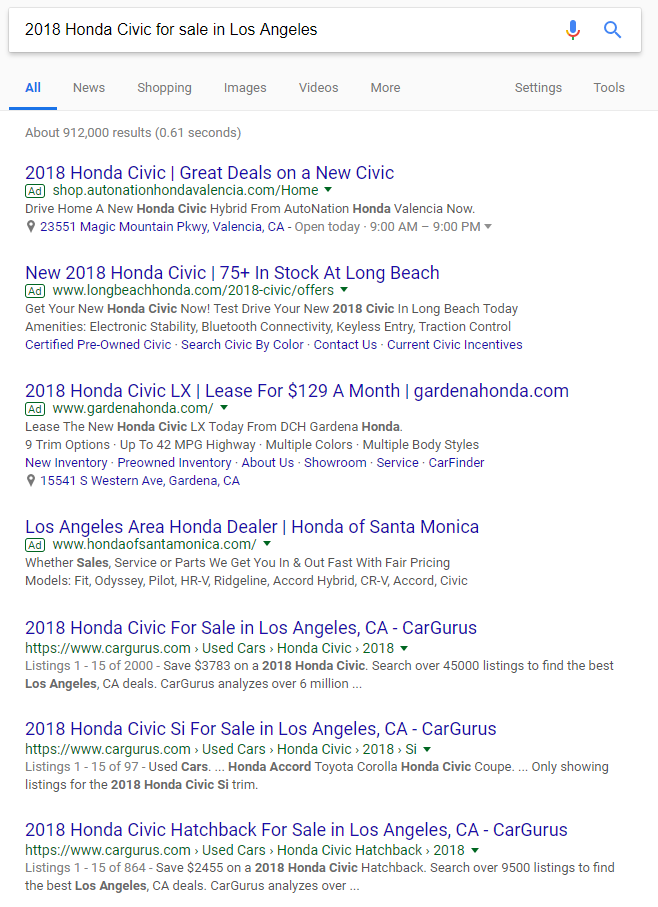The image is a cropped screenshot of a Google search page, focusing on the search results for "2018 Honda Civic for sale in Los Angeles." The Google logo, browser tabs, and navigation elements have been excluded from the screenshot.

In the search bar, the query "2018 Honda Civic for sale in Los Angeles" is visible. Below the search bar, the top entry in the search results lists "2018 Civic - Great Deals on a New Civic." To the left of this entry, there is a green box labeled "Ad." To the right, the website "AutoNation Honda Valencia" is indicated, followed by its URL: "shophonda.AutoNation.com." A brief description of the website is provided, and at the bottom of this listing, there is a location icon next to an address displayed in blue, along with information about the business hours.

The second entry is also marked as an ad and is from "Long Beach Honda." The third entry, another ad, is from "Gardena Honda." The fourth ad-listed entry is from either "HondasofAmerica.com" or "HondasofSantaMonica.com."

Following the advertised results, there are organic search results from "cargurus.com." The first non-ad result is from "CarGurus," followed by another CarGurus entry, and the final listing is also from CarGurus, all of which are not advertisements.